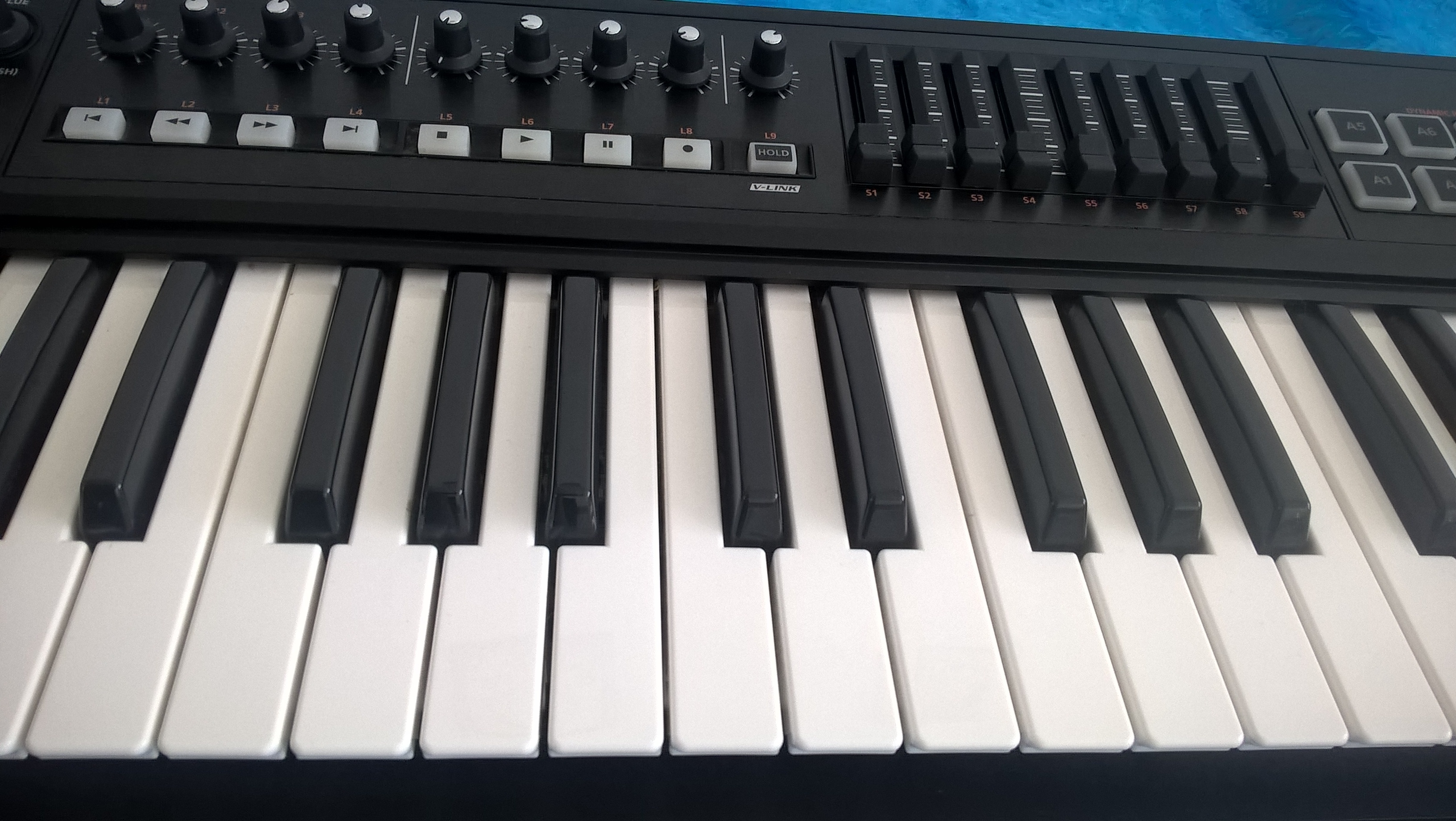The image depicts an electronic keyboard with a variety of controls and features. The top part of the keyboard is black, while the front showcases the traditional white and black keys - the longer keys being white and the shorter ones black. At the bottom edge of the keyboard, there is a black lip.

On the left side, there are nine black knobs, each marked with white line dots around them. Below these knobs are white buttons featuring black symbols for fast forward, play, pause, and stop. In the center of the panel, there are approximately nine sliders with white lines on either side for accurate adjustments.

To the right side of the control panel, there are four off-white squares, each containing a smaller black square inside. These could be pads or additional buttons. This detailed arrangement highlights the complexity and functionality of the instrument.